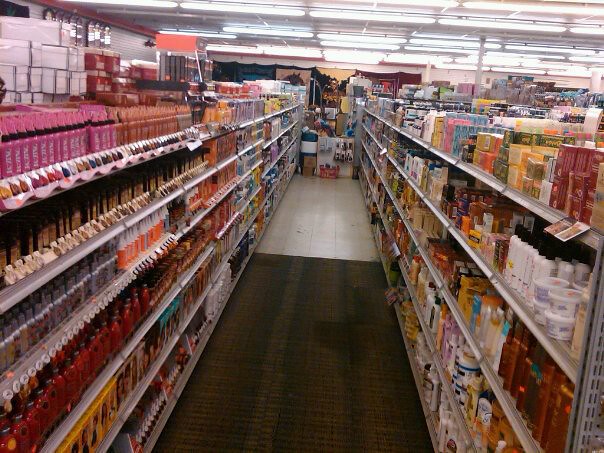This photograph captures the interior of a retail store, likely specializing in cosmetics and beauty products. The image focuses on the middle aisle, flanked by well-stocked shelves on both sides. Each shelf is brimming with numerous bottles, predominantly labeled with pink and red, suggesting a collection of women’s beauty products and toiletries. The scene has a nostalgic quality, as if taken with a point-and-shoot camera from the early 2000s. The store's layout and aesthetic differ subtly from typical U.S. retail environments, hinting that this might be a location outside the United States. The visual details, combined with the slightly aged photographic tone, evoke a sense of browsing through a vintage beauty emporium.